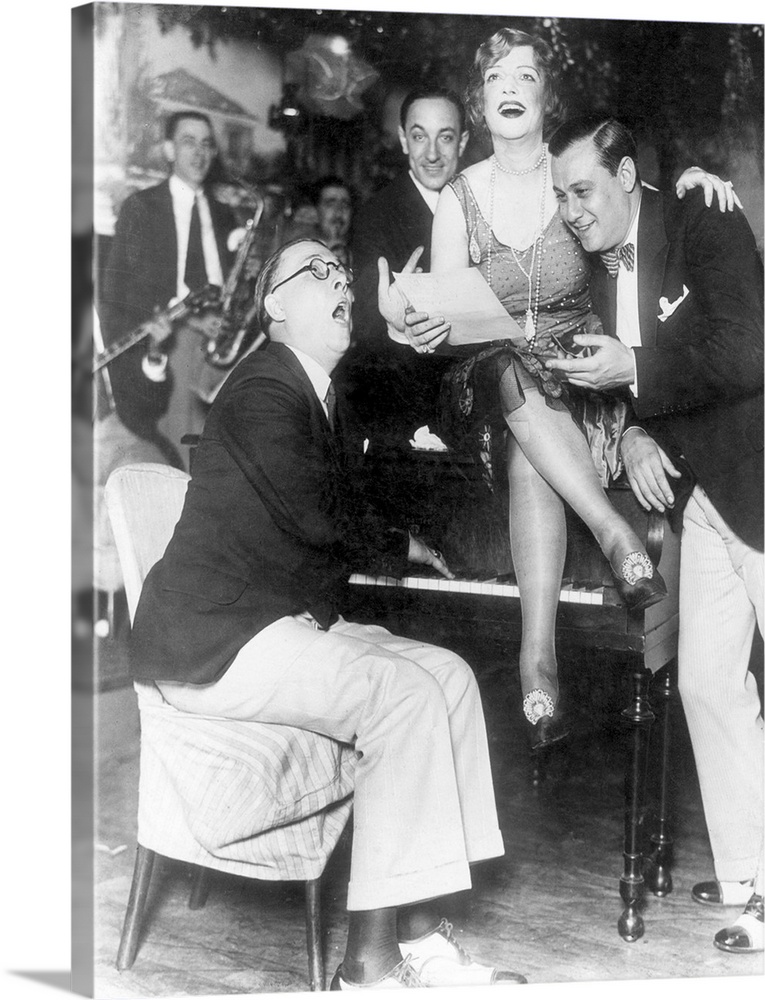In this evocative black and white photograph reminiscent of the Prohibition era, a lively scene unfolds against the backdrop of a sophisticated club or restaurant. Center stage is a polished band, featuring a guitarist and a saxophonist, all impeccably dressed in suits and adding a rich musical ambiance. On the left, a distinguished pianist is captured mid-performance, his fingers dancing across the keys of a piano. He sports a black blazer, tie, light-colored pants, and black and white dress shoes, his expression animated as if singing.

Seated with elegant poise atop the piano is a woman with short, wavy hair styled in a bob, adorned in a low-cut, tank top-style dress and a long, beaded pearl necklace. She holds a sheet of paper, likely the lyrics, and her graceful legs are crossed. She wraps her left arm around a dapper man beside her, who shares in the musical moment. This man mirrors the piano player's attire and adds to the charm with his bow tie.

Together, their gazes and expressions suggest a shared song, creating a harmonious tableau. Behind them, the smiles and the instruments of other band members — perhaps playing guitar and saxophone — further enrich the scene, hinting at a vibrant, bygone entertainment milieu.